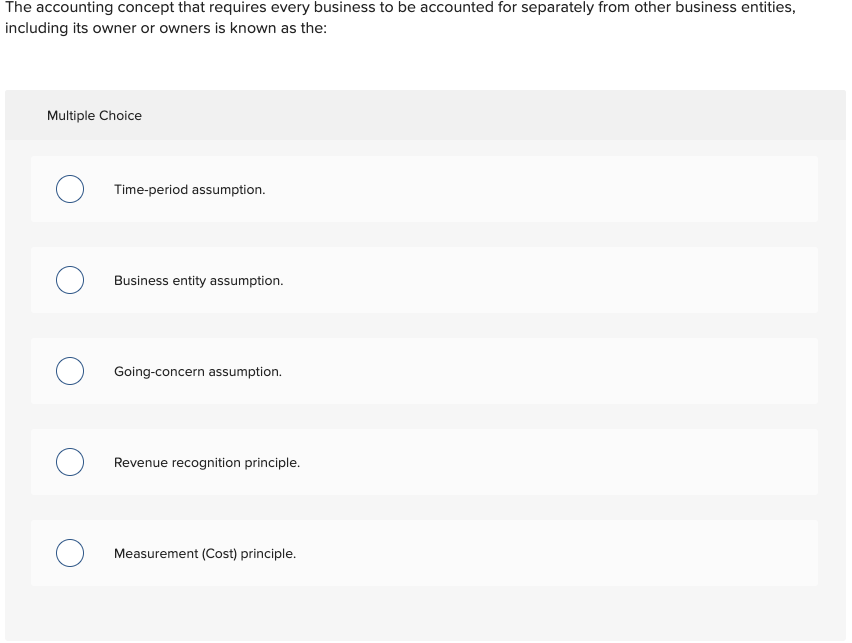The screen features a shades-of-gray theme with a darker gray banner at the top that reads "Multiple Choice" in black text. Below this banner, the background transitions into a lighter gray, containing five lengthy, light gray rectangles arranged vertically. Each rectangle contains a small, white, clickable circle set against a blue background, designed for multiple-choice selection. The text within these rectangles is uniformly in black, and they read as follows:

1. "Time Period Assumption"
2. "Business Entity Assumption."
3. "Going Concern Assumption."
4. "Revenue Recognition Principle."
5. "Measurement (Cost) Principle."

The overall style is neat and blocky, with a highly organized layout. Each clickable circle suggests an interactive element, allowing users to select their answer from these predefined options.